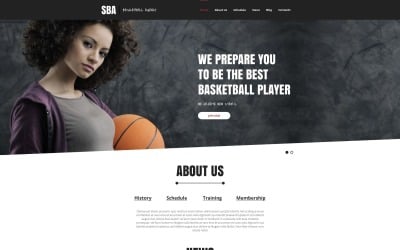This color photograph is a screenshot of a website featuring a young female basketball player. The background of the image is a dark gray, creating a striking contrast. At the top of the picture, there's a solid black rectangular bar with "SBA" prominently displayed in large white letters. In the center of the photograph, the bold statement "We prepare you to be the best basketball player" is written in sizeable white letters, catching the viewer's attention. Below this, there is a solid white filled oval, which serves as a focal point directing to the next segment of the site. 

Further down in the screenshot, against a white background, are black text navigation options: "About Us," "History," "Schedule," "Training," and "Membership." Below these links, there is additional small text that is not clearly visible. The screenshot itself is rectangular, with the long side being horizontal. The young female basketball player, who is positioned slightly to one side, has curly hair and is confidently holding a basketball under her left arm. Her presence on the website highlights the focus on empowering and training athletes.